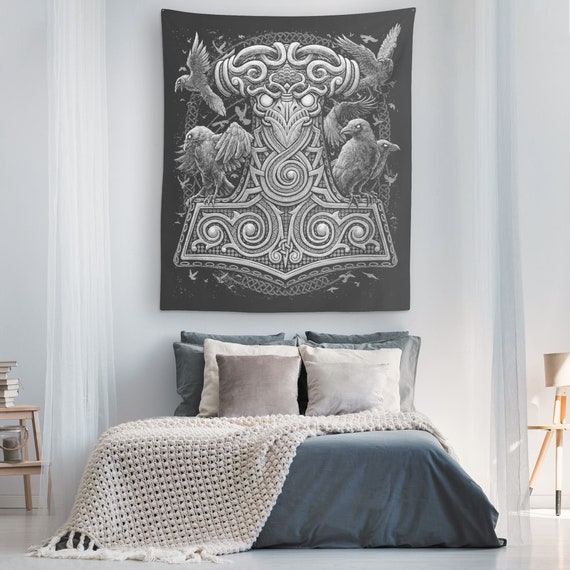The image features a meticulously arranged bedroom with white walls and a blue-themed decor. The bed, adorned with a slate blue comforter and a white knitted spread, is topped with eight pillows in varying shades of blue, white, and gray. Above the bed hangs a striking black-and-white poster, or perhaps a tapestry, displaying an intricate 2D drawing of a bird that resembles a rooster or a crow. The bird’s detailed design is filled with ornate swirls and geometric patterns, giving it an almost relic-like appearance. The bird’s eyes, beak, and outline are distinct, while additional crows with menacing empty eyes are interwoven into the design. The room is framed by two sheer curtains on the back wall, adding a touch of elegance. To the left of the bed, a side table holds a stack of books and a canister, while the right side table features a lamp. Light streams in from the right, hinting at a window just outside the frame. A subtle touch of sunlight enhances the cozy ambiance of the room.